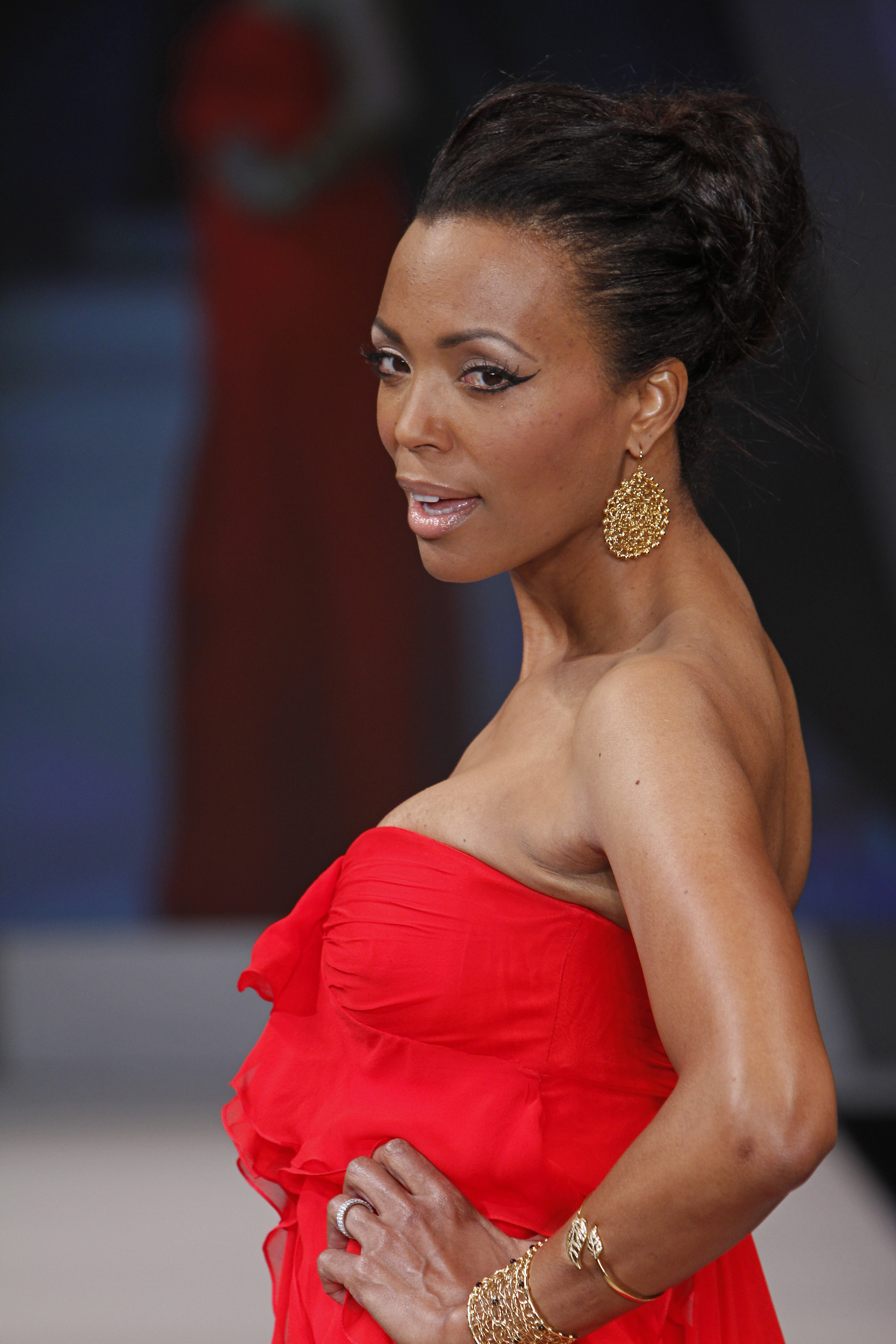The image is a detailed photograph of a woman, who resembles a movie star, captured at what appears to be an official gala event. The woman is wearing an elegant red dress that barely covers her breasts, giving the impression they are slightly squeezed by the top. The dress looks light and silky with significant volume. Her accessories include striking golden earrings, a sophisticated leaf-patterned open-ended golden bracelet, and several ornate bangles on her left wrist, along with a ring on her finger. Her hairstyle is an elegant updo, enhancing her glamorous appearance. The background is notably blurred, making it hard to decipher specific details; however, hints of white, gray, and blue are visible, possibly including blue stairs. There also seems to be a red vertical shape that could be another attendee in a red dress. The overall focus remains sharply on the woman, accentuating her poised and radiant presence.